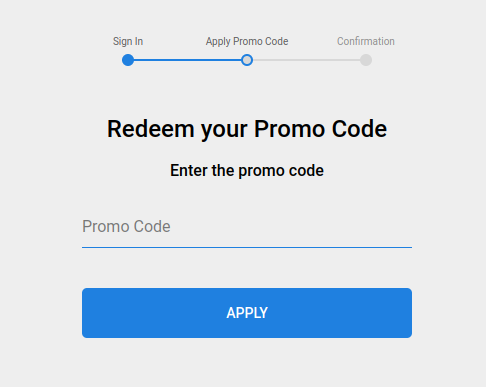In the image, a light gray square serves as the backdrop, drawing attention to a multi-step process for redeeming a promo code. On the left side of the square, a textual label "Sign In" is placed, guiding users towards the first step of the process. Beneath this label is a blue circle connected to a blue line, which culminates around a gray circle. This gray circle is marked with "Apply Promo Code" above it, visually representing the subsequent step.

Proceeding rightward, there's a gray line extending to a gray circle, where it displays "Confirmation" in lighter gray text, indicating the final step. Positioned centrally beneath the "Sign In" and "Confirmation" markers, the instruction "Redeem Your Promo Code" appears in bold, darker print with each major word capitalized.

Below these phases, centrally aligned, the phrase "Enter the Promo Code" is presented in darker print, commanding user attention. Directly under this phrase is an empty blue input line, labeled with the faded gray text "Promo Code."

At the bottom of the image, a prominent dark blue clickable banner stands out. In the center of the banner, the word "Apply" is displayed in bright white text, inviting users to proceed with their promo code application.